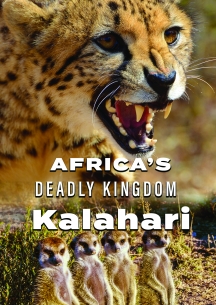The image is an artistic and detailed front cover for a magazine or advertisement titled "Africa's Deadly Kingdom: Kalahari." Positioned centrally in bold white text, the title is divided into three distinct fonts: "Africa's" in one font, "Deadly Kingdom" in another, and "Kalahari" in yet another style, emphasizing its importance. Dominating the top half of the image is a majestic cheetah (possibly mistaken for a leopard), with its striking orange and white fur, piercing red eyes, and snarling mouth open, displaying sharp teeth and whiskers. This fierce predator appears to be gazing into the distance, perhaps in search of prey. Below, the image transitions to four meerkats standing upright on their hind legs, exhibiting their characteristic alert and cautious posture. The meerkats, although somewhat blurry, can be identified by their distinctive black facial markings and curious expressions. They stand amidst tall grasses, further enhancing the authenticity and depth of the Kalahari habitat depicted in the cover. The entire image is rendered in vivid color, highlighting the contrast between the powerful predator and the vigilant prey within this harsh, dramatic African landscape.